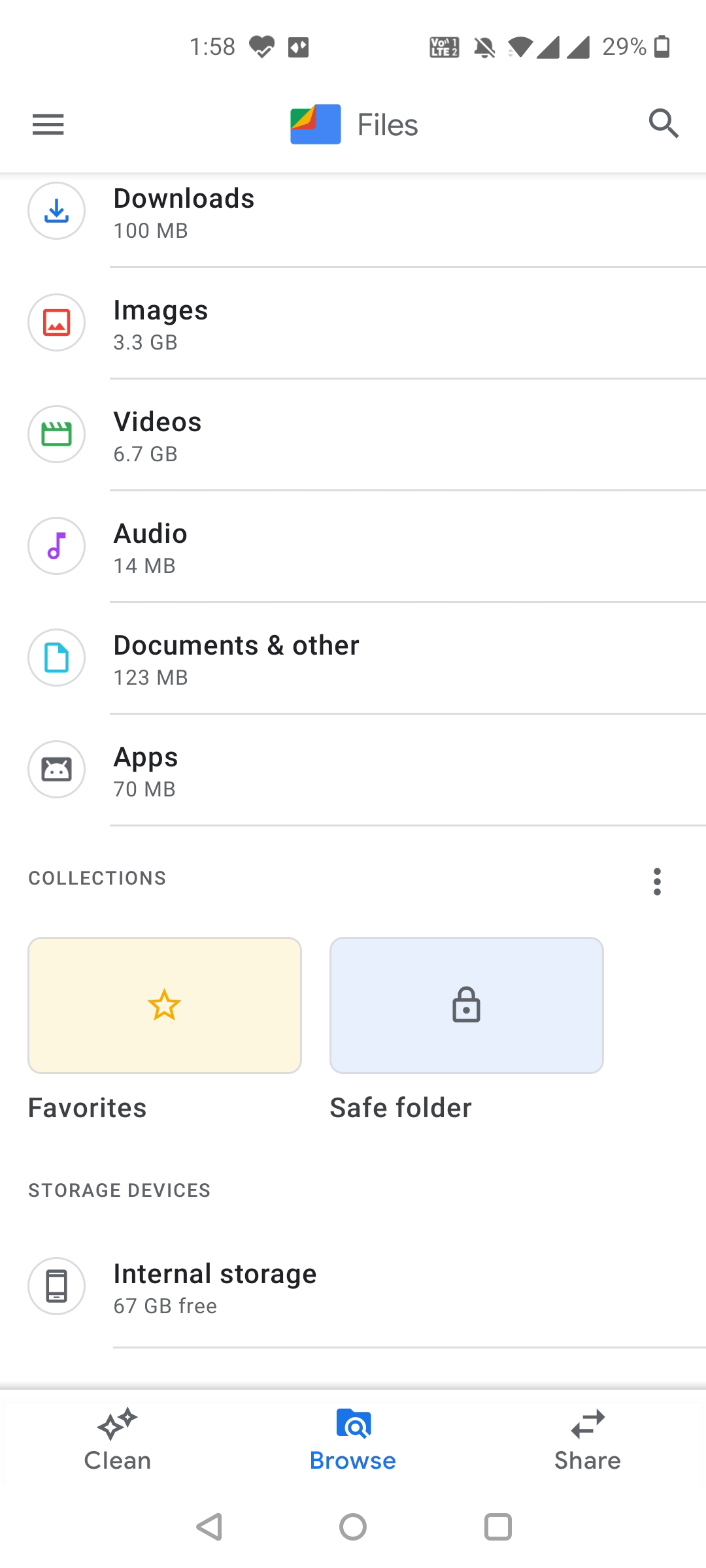The image depicts a smartphone interface in a vertical format, displaying the current time at 1:58 PM in the top left corner. Adjacent to the time, icons for heart, battery (at 29%), and Wi-Fi reception are visible. Below the status bar, the screen is titled "Files," with a blue folder icon beside the title, accompanied by a three-line menu icon on the left and a magnifying glass search icon on the right.

Under the "Files" title, several categories are listed:
- **Downloads:** 100 MB, denoted by a blue downward arrow within a circle.
- **Images:** 3.3 GB, represented by a red landscape icon.
- **Videos:** 6.7 GB, indicated by a green video icon.
- **Audio:** 14 MB, shown with a purple music note icon.
- **Documents & Other:** 123 MB, depicted by a blue page icon.
- **Apps:** 70 MB, marked by an Android icon.

Further down, the "Collections" section features two categories:
- **Favorites:** Identified by a yellow box with a star.
- **Safe Folder:** Marked by a blue icon with a small lock.

At the bottom, "Storage Devices" mentions internal storage availability, showing 667 GB free. The interface also includes options at the very bottom for "Clean," "Browse," and "Share."